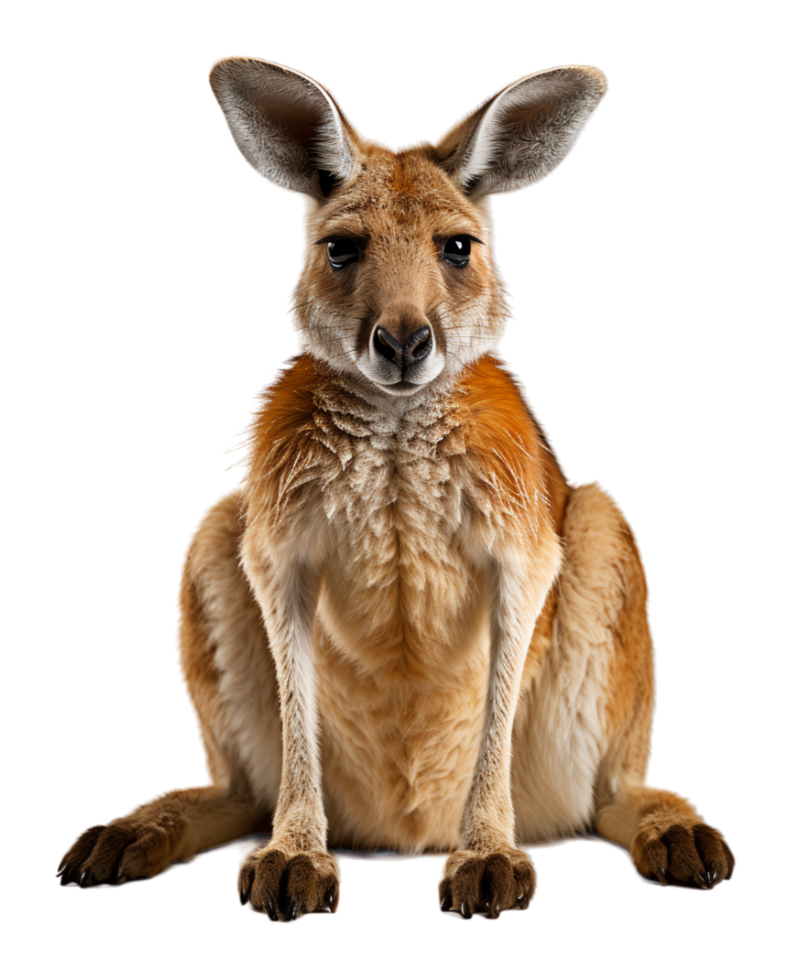In this detailed photograph, a creature resembling a large bunny or a young kangaroo is centered against a pristine white background. This tawny brown animal, with its golden amber fur, is poised on its hind legs with its long, thin front arms extended forward. The creature has large, dark brown eyes accented with very prominent eyelashes or eyelids, and a black nose framed by long, black whiskers. Its underbelly and the area under its nose and cheeks are coated in a lighter, creamy beige fur. The ears, which are long, hairy, and grayish in color, stand erect above its head. The tips of its paws and the toenail areas display a deep dark brown hue. Despite the conflicting interpretations of the animal, its striking, almost whimsical appearance remains a captivating feature of this well-composed image.